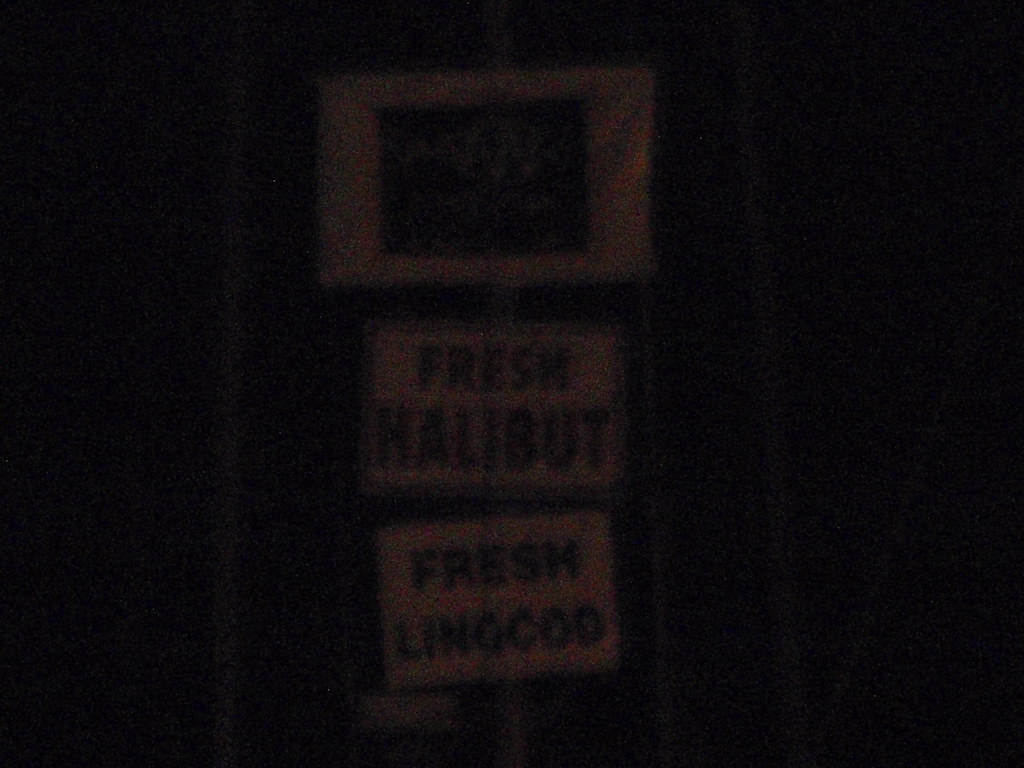The image is a very low-resolution and dark photograph, likely taken at night with a camera that does not perform well in low light conditions. The picture is predominantly black, with indistinguishable background details. Centrally, there are three vertically aligned white signs, appearing to be mounted on a pole or possibly a door frame or wooden paneling. The top sign has a white border with an unclear central dark image or text, hinting it might feature the name of a business, possibly related to seafood. The middle sign distinctly reads "FRESH HALIBUT" in bold black letters, and the bottom sign, also in bold black letters, reads "FRESH LINGCOD." The layout and clarity of the middle and bottom signs suggest they are well-defined against the dark backdrop. White streaks or potential lens flare are visible in the middle of the photograph, adding to the visual noise and ambiguity surrounding the setting and specifics beyond the illuminated signs.